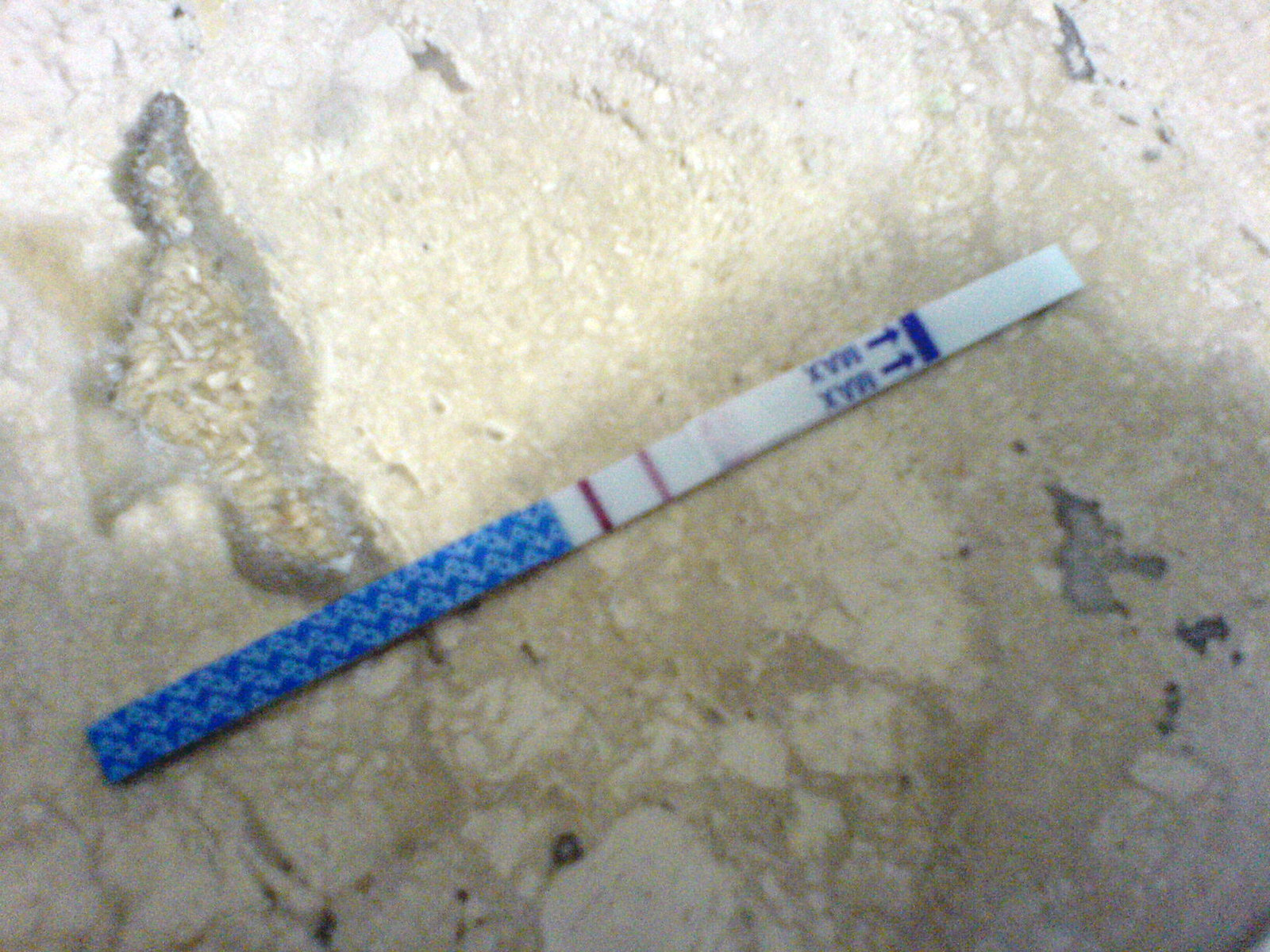This horizontal, rectangular image is slightly blurry, and there's a noticeable spread of light that starts at the middle of the left edge, extending diagonally to the top left corner, crossing over to the top right, and then descending slightly on the right and in the middle. This light creates a brightness that obscures some details and the exact nature of the scene. The main background of the photograph is cream-colored, though it appears disrupted by a few brown spots that might indicate cracks in the stone or cement.

Prominently featured is a very thin, rectangular object, resembling a COVID-19 testing strip, positioned diagonally with one end pointing to the upper right and the other to the lower left. The lower left portion of this strip, which takes up almost half of it, is royal blue with a small blue design. The upper right end is white. In the strip's middle segment rests a royal blue rectangular block, strategically placed with two arrows pointing towards it. The arrows, which originate from the bottom right, direct attention to this block towards the upper left.

To the left of the arrows, the word "MAX" is written twice, aligned vertically, as if viewed from the upper left corner. The test strip transitions to white again, leading to a section marked by two magenta or hot pink stripes. One of these stripes is a deep, bold color, while the other is lighter but still distinctly visible.